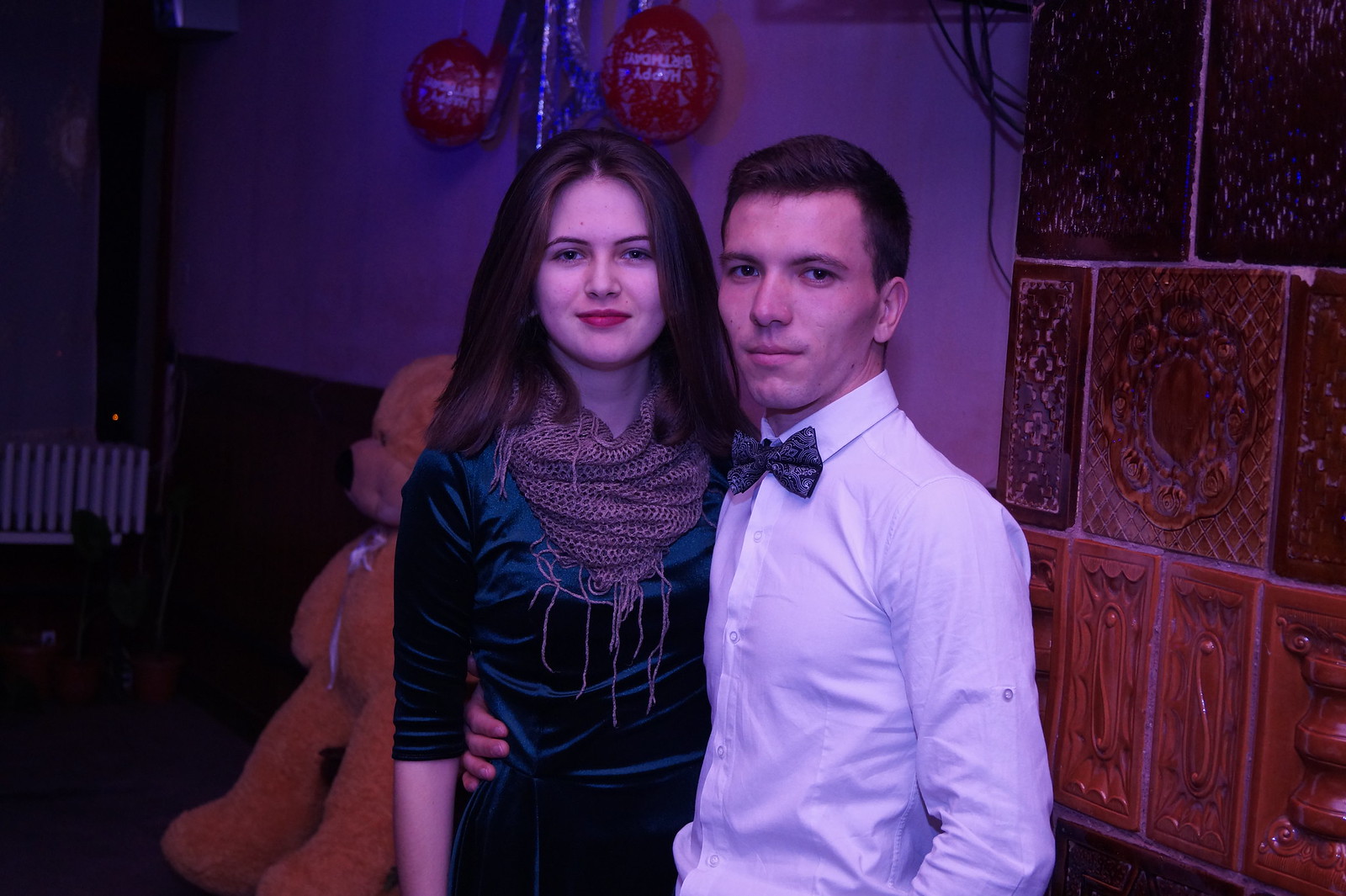The photograph captures a dimly lit interior setting featuring a man and a woman posing together against a white wall adorned with intricate, mosaic-like tiles, some of which are red. On the left, the woman with long brown hair and red lipstick is elegantly dressed in a velvet blue dress with elbow-length sleeves, accessorized with a knit brown scarf. Beside her on the right, the man with short brown hair and brown eyes is wearing a white button-up shirt, a black bow tie with white designs, and has his hand around her waist. Complementing the scene, a large, human-sized yellow teddy bear sits on a chair to their left, while two upside-down balloons above them spell out "Happy Birthday" in white text.